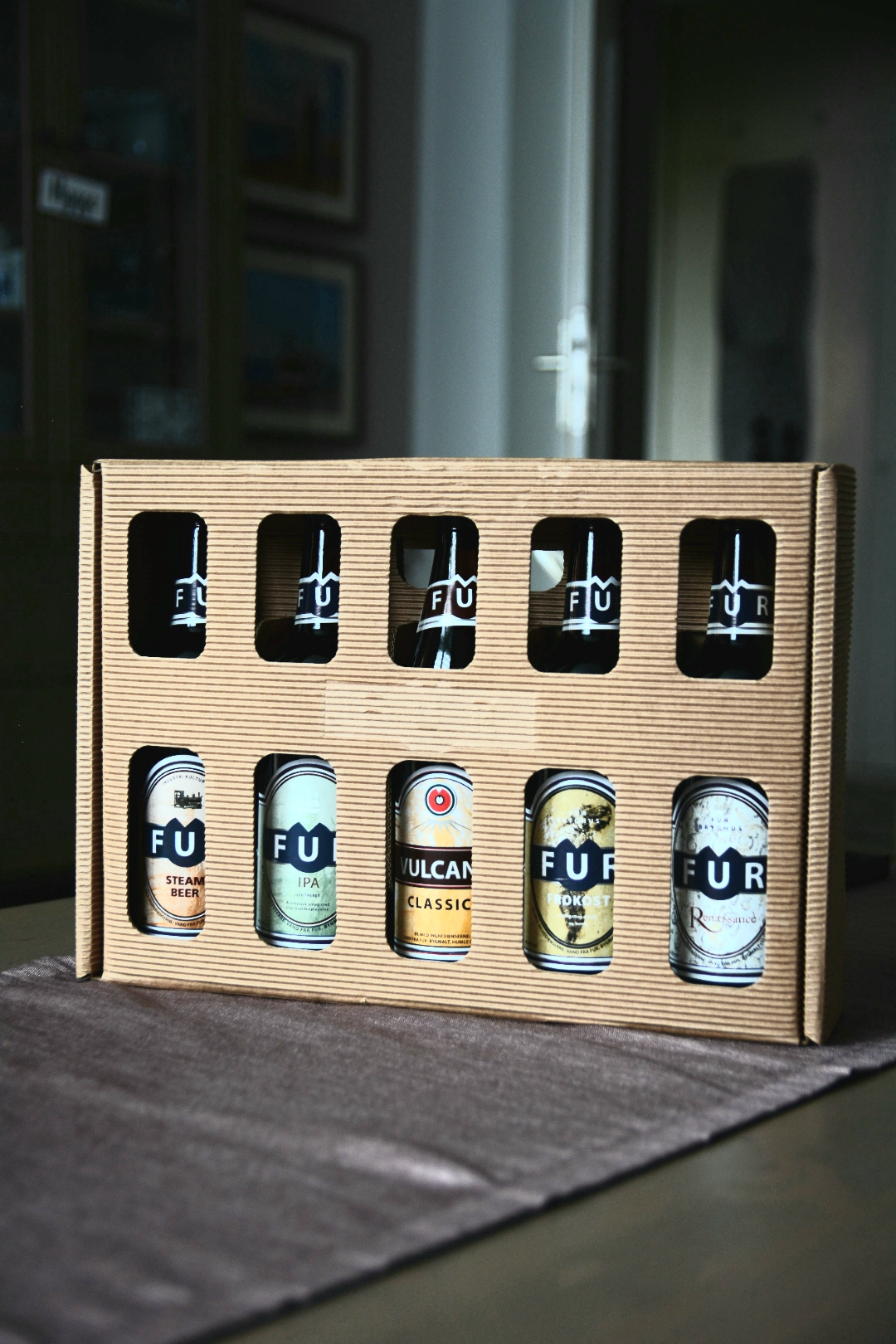This photograph depicts a brown cardboard box characterized by horizontal dark and light brown lines. The box is designed with rectangular cutouts through which five glass bottles are visible. The bottles are adorned with white labels that display the partial writing "FUR." Each bottle has additional colored labels around the neck, presenting hues of pink, green, orange, yellow, and white. 

The cardboard box, which opens from the top or bottom, sits atop a dark grey or silverish dark grey table surface, potentially lined with a table liner. The table itself appears to be a very dark brown wood. In the background, there are blurred elements, including walls with square or rectangular paintings, a door with a silver handle to the left, and a glass case containing various items.